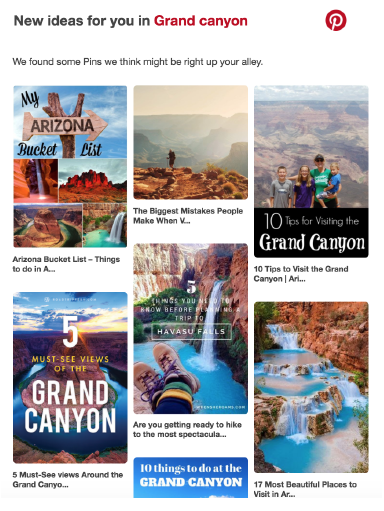Here is a detailed and cleaned-up caption for the image:

"This collage from Pinterest, titled 'New Ideas for You in Grand Canyon,' showcases various inspiring visuals related to exploring Arizona. Among the images is a signpost reading 'My Arizona Bucket List,' featuring a wooden arrow labeled 'Arizona' pointing to the right. The collage includes picturesque waterfalls and a shot of a hiker in a secluded area, accompanied by the truncated text 'The biggest mistakes people make when...'. Another image shows a mother posing with her three children under the caption '10 Tips for Visiting the Grand Canyon.' Additionally, there's a breathtaking view of the Grand Canyon surrounded by water, titled 'Five Must-See Views of the Grand Canyon.' The final image provides practical advice with 'Five Things You Need to Know Before Planning a Trip to Havasu Falls,' depicted alongside a close-up of someone's boots resting near a waterfall."

Feel free to adjust the level of detail or specific focus as needed for your purpose!